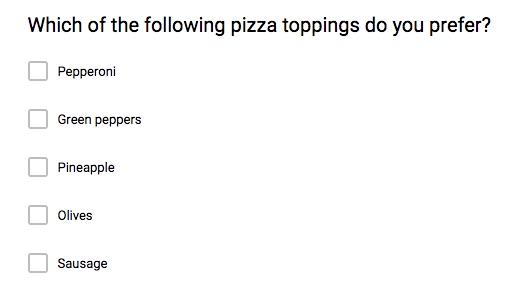The image displays a clean, minimalist survey form set against a white background. At the top center, there is a bold, black text header that reads, "Which of the following pizza toppings do you prefer?" Below this question, there is a list of five pizza topping options: Pepperoni, Green Peppers, Pineapple, Olives, and Sausage. Each option is accompanied by a small, light gray checkbox to the left, indicating areas where respondents can select their preferred toppings. The simplicity of the design focuses attention solely on the topping choices, making the survey straightforward and easy to complete.